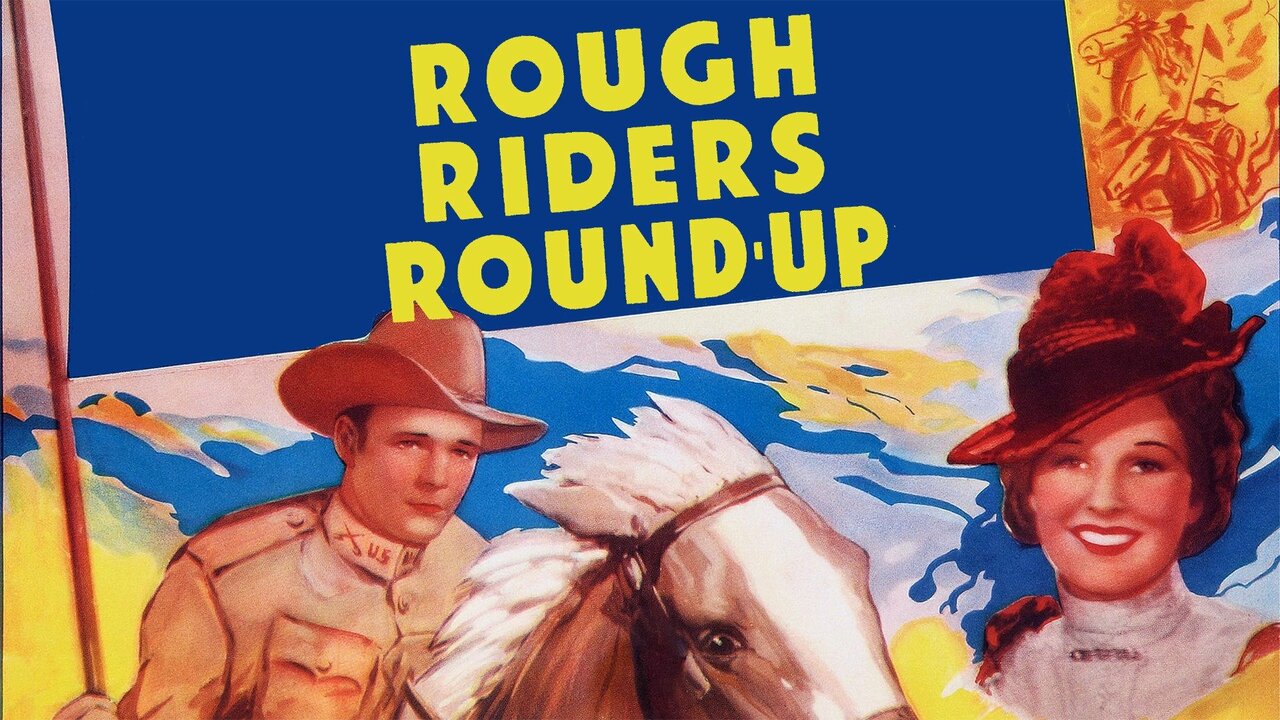The image depicts an old recruitment poster titled "Rough Riders Round Up." At the top, a blue flag with bold yellow text announces the title. The flag is attached to a reddish stick held by a man in a military uniform. The man, who is Caucasian, wears a brown cowboy hat and a tan or brown jacket with "U.S. Army" markings, including collar insignia that appear to be crossed swords. He is riding a dark brown horse with a white mane and a white stripe down its head.

To the bottom right, there is a partial view of a woman with a big smile, white teeth, a red hat with a bow, and red lipstick. She's dressed in a high-necked, lacy white shirt, reflecting a style from the late 1800s or early 1900s. 

In the background, there are illustrations of other cowboys on horseback, some holding flags. The scenery behind features a blend of blues, yellows, and oranges, suggesting a dynamic sky and possibly a mountainous terrain. The overall composition with the man on horseback, the prominent flag, the woman, and the detailed background illustrates a vibrant and patriotic recruitment scene.